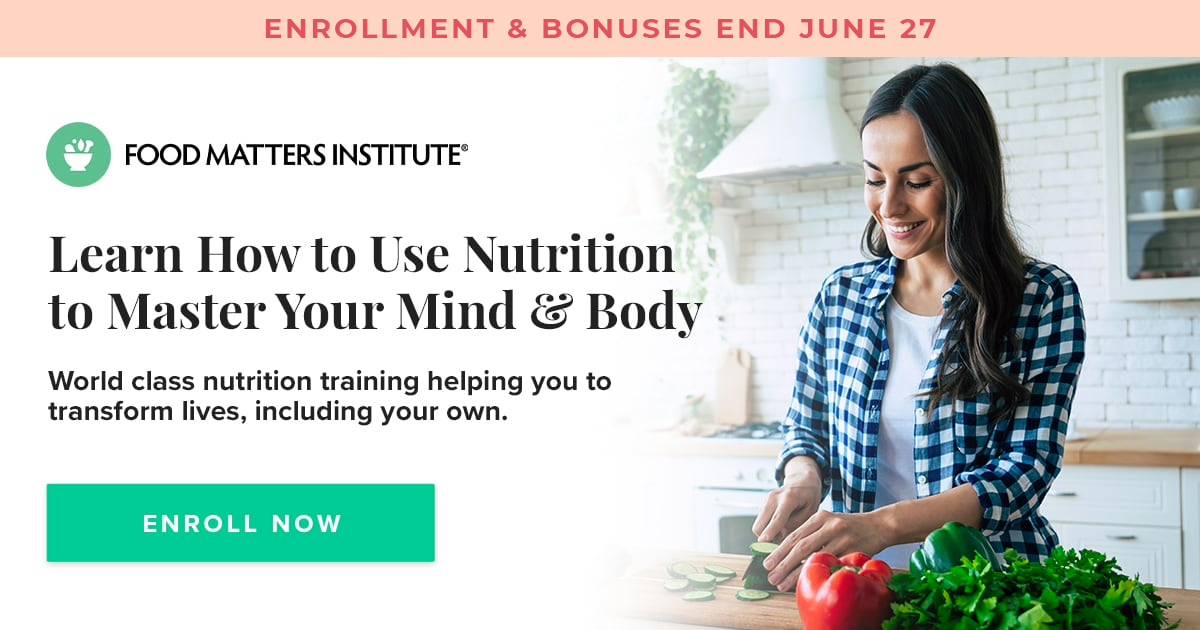This vibrant promotional image features a compelling message regarding an enrollment deadline. The top section of the image showcases a light pink background with red text stating, "Enrollment and bonuses end June 27." On the left side, a prominent white background contains black text associated with the Food Metas Institute. The institute’s logo, situated at the upper left corner, features a white icon of a mortar and pestle within a green circle. Below the logo, a motivational message invites readers to "learn how to use nutrition to master your mind and body," followed by an assurance of the institute's "world-class nutrition training to help you transform lives, including your own." Additionally, a green button with the phrase "Enroll Now" in white text calls for immediate action. 

On the right side of the image, a cheerful woman in a white and blue t-shirt, with a white vest over it, is depicted happily chopping a cucumber on a brown table. The fresh cucumber is being sliced with a knife, amidst an array of colorful vegetables including a green bell pepper, a red bell pepper, and green spinach leaves. The scene is set in a kitchen environment, with a white table and white cabinets in the background adding to the clean, fresh atmosphere. This engaging image perfectly combines informative text with a lively visual, designed to capture interest and prompt immediate participation in the Food Metas Institute's nutrition program.